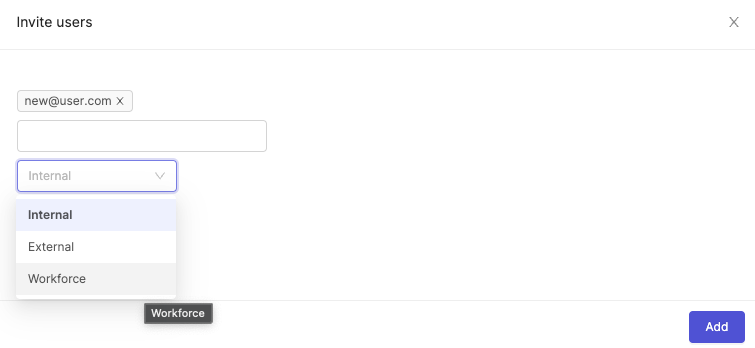The image depicts an "Invite Users" page for a program or app with a minimalistic design on a white background, featuring ample white space. 

At the top left of the page is the title "Invite Users," while the top right corner has a gray "X" icon for closing the page. Below this section lies a thin gray horizontal line serving as a divider. 

On the left side, a column features various input fields for information. The first box, outlined in a light gray, contains the email address "new@user.com" with an "X" icon for canceling the entry. Below this, there's an empty text box ready for input. 

Further down is a drop-down menu, currently highlighted with a purple outline, indicating the option "internal" in gray text. When expanded, three options are displayed with different background shades: "internal" in bold text with a light shade of purple, "external" with a white background, and "workforce" with a light gray background.

The bottom of the page is separated by another thin horizontal line, below which two action buttons are positioned. On the left is a dark gray button labeled "Workforce" with white text. In the bottom right corner is a purple "Add" button featuring white text and rounded corners.